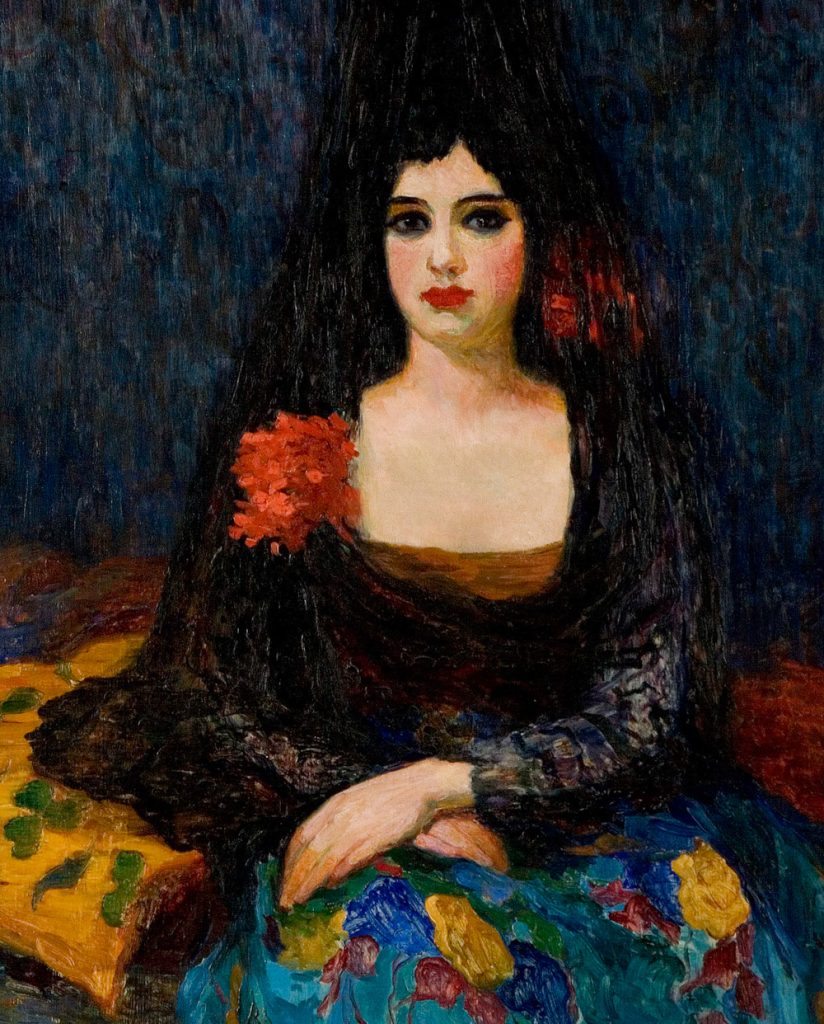The painting depicts a young, light-skinned woman with dark black hair adorned with a red ribbon on the left side of her head. Her complexion is very pale, almost white, with defined black eyebrows, dark eyeliner, and strikingly red lips. Her cheeks are accentuated with red blush. The woman is adorned in a dark covering that appears to be a shawl, with a brownish undershirt visible above her chest. Red flowers are positioned near her left shoulder and possibly woven into her headdress.

She is seated with her large hands resting on her right thigh, one overlapped atop the other, against a backdrop that features a mix of blue, black, and reddish hues. The lower part of her attire consists of a flowing dress skirt, embellished with an array of indistinct yet vividly colored flowers in shades of blue, yellow, and red. The seat she occupies is covered with colorful blankets, primarily yellow with green clovers, blending into shades of red, blue, and green on the left side. Her posture is upright, gazing directly at the viewer, suggesting an air of quiet confidence or contemplation.